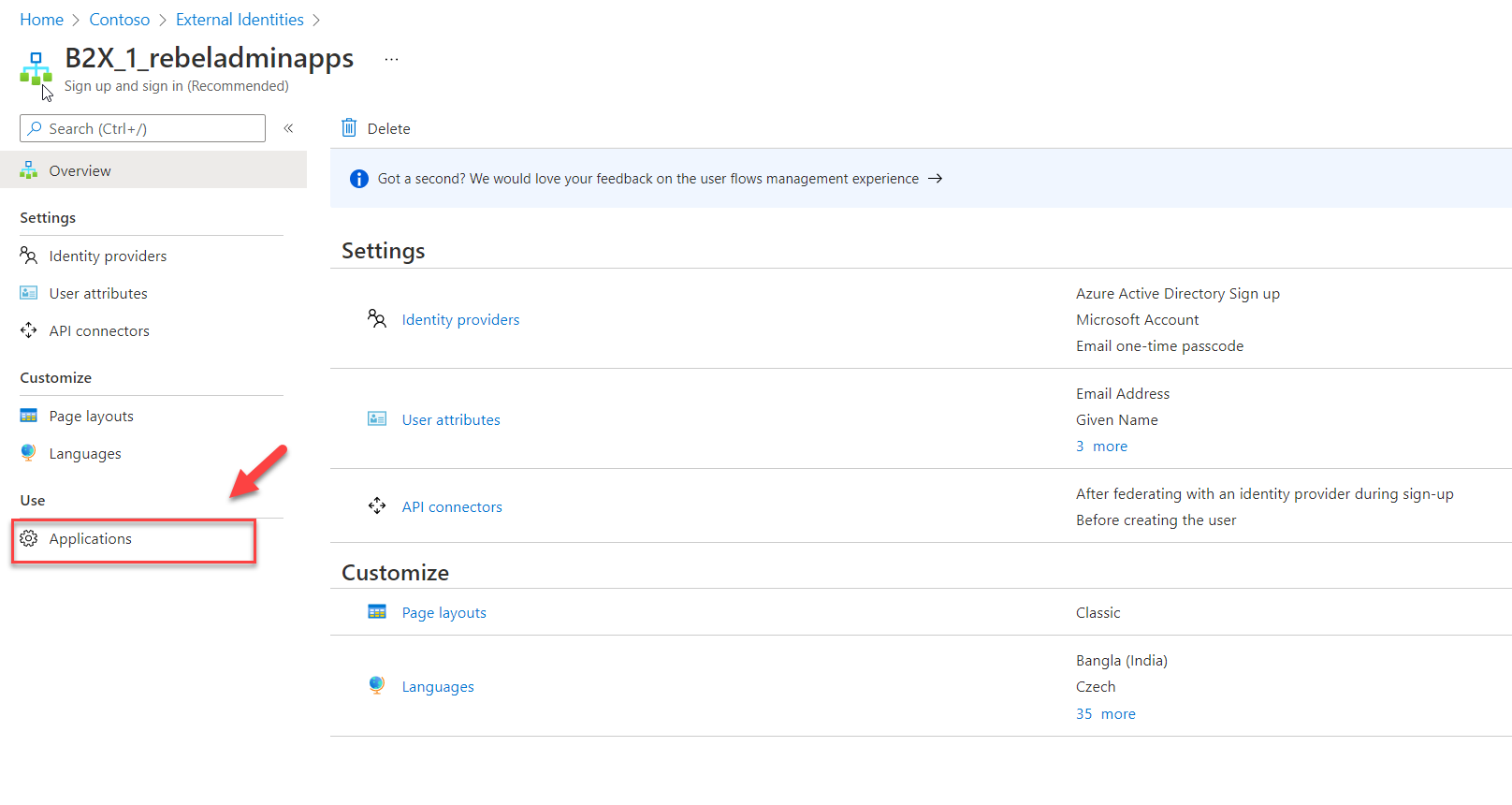The image displays a webpage with a structured navigation menu and various interactive elements. At the very top, the navigation bar features options labeled "Home," "Contoso," and "External Identities." Just below this header, the page title reads "BTX_one_rebeladminapps," accompanied by prompts for "Sign up" and "Sign in" under the "Recommended" section.

On the right-hand side, a search box with a blue magnifying glass icon is prominently positioned. The page also includes an "Overview" button for a broad overview of the content.

Several sections with different settings are presented on the page. The main settings category includes "Identity Providers," "User Attributes," and "API Connectors." Highlighted within a red box and indicated by a red arrow is the 'Applications' setting under the "Use" category, marked by a gear icon. 

Further customization options are available under a section titled "Customize." This section features "Page Layout" with a calendar icon, and "Languages" with a globe icon. Clicking on "Page Layout" shows options like "Classic." Under "Languages," the page lists "Bangla" and "Czech," along with an additional "35 more" other languages, accessible via a blue button.

The design of the page predominantly features a white background, interspersed with sections of blue and black text, lending it a clean and organized appearance.